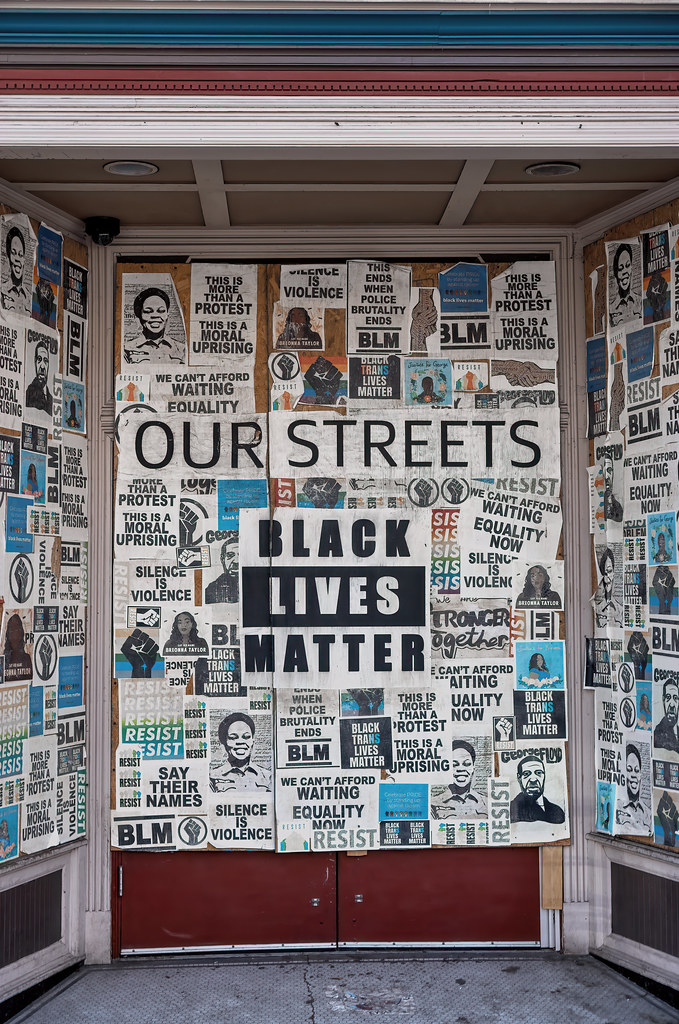This photo depicts a heavily postered entryway, possibly a storefront or a building entrance, covered with a diverse array of protest flyers centered around the Black Lives Matter (BLM) movement. In the heart of this assemblage, a prominent Black Lives Matter logo stands out, surrounded by powerful slogans including "This is more than protests, this is a moral uprising," "We can't afford waiting, equality now," and "This ends when police brutality ends, BLM." Additional messages like "Silence is violence" and "Black Trans Lives Matter" add to the chorus of demands for justice. Amongst these flyers are images of Black individuals, notably including George Floyd, whose tragic death sparked widespread activism, along with unnamed women who also symbolize the movement's struggle. The entire space is layered with similar protest visuals, creating a tapestry of resistance and solidarity. A prominent white banner with a simple, thin, sans serif black font reading "Our Streets" spans the top, anchoring the amalgamation of boldface, sans serif messages that emphasize unity in the face of ongoing social and racial injustices. The image is tightly framed, honing in on these impactful messages and obscuring the possible doors and display windows underneath the posters.